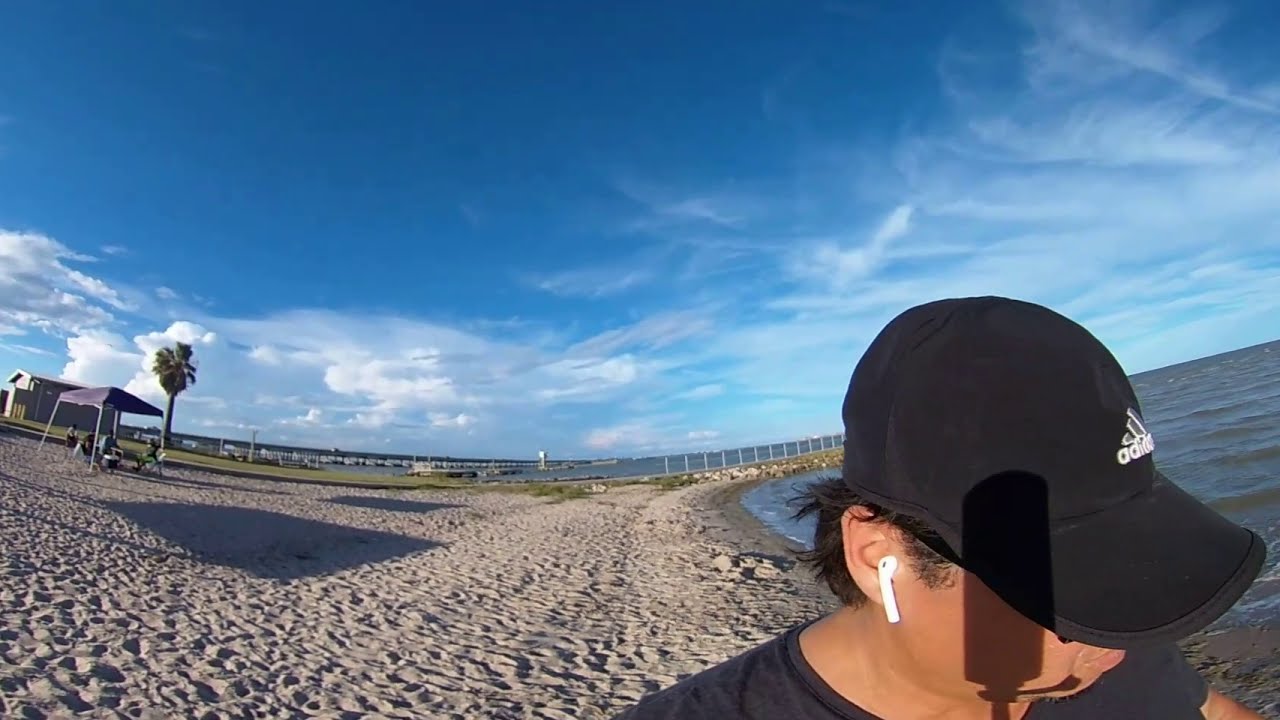The photograph is a slightly fisheye-lensed selfie of a young man taken on a beach. He occupies the bottom right corner of the image and is visible from his top shoulders to the top of his head. The man is clad in a black, short-sleeve t-shirt and a black Adidas baseball cap emblazoned with the logo in white. He has white wireless earbuds in his ears and is looking downward, towards the bottom right corner of the frame. His dark hair and slightly heavyset appearance are partially discernible.

The upper half of the photograph is dominated by a light blue sky interspersed with large white clouds, while the bottom half showcases a sandy beach extending behind the man. The sand, appearing heavily trodden and a mix of white-tan and gray hues near the waterline, stretches leftward toward a red canopy tent equipped with seats, possibly occupied by people. Further left, a palm tree and additional beach structures are faintly visible. To the right, greenish ocean water laps at the shore. The image, capturing the late evening ambiance, also reveals the shadow of the man's smartphone on his face, suggesting the use of a selfie stick to take the photograph.